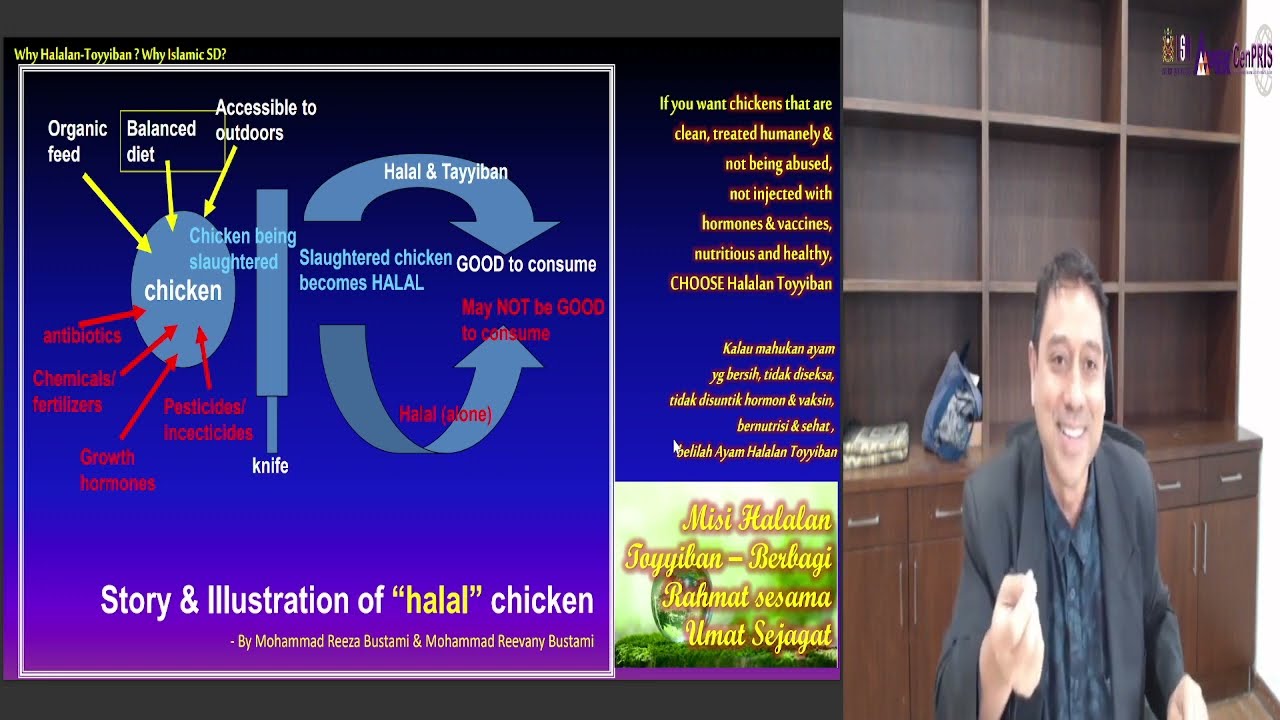The image is divided into two sections side by side. On the left, there is a detailed PowerPoint-style presentation with a gradient background transitioning from dark blue at the top to light blue with some purple. At its core, the visual exhibit focuses on the pros and cons of consuming halal chicken. A central blue circle with the word "chicken" is surrounded by yellow arrows at the top labeled "organic feed," "balanced diet," and "accessible to outdoors." Red arrows pointing to the chicken, but these are hard to read against the background. Near the bottom, a gray vertical line with the word "knife" sits beside a comprehensive illustration and narrative of halal chicken by Muhammad Riza Bustami and Muhammad Referee Bustami. The bottom contains various languages and additional text in yellow and red. Informational content mentions the benefits of choosing halal chicken, stating attributes like humane treatment, hormone-free, and nutritious features.

On the right side of the image, a man stands smiling in front of a wooden cabinet comprised of several square compartments. Dressed in a black jacket and blue buttoned-up shirt, he has dark black hair, brown eyes, and light skin. His posture includes one hand on the table in front of him and the other raised with curled fingers. Behind him on the table, there's a bag filled with a white substance and a blue piece of paper. The overall setting likely represents a comprehensive presentation blending text and visuals, similar to a PowerPoint format.